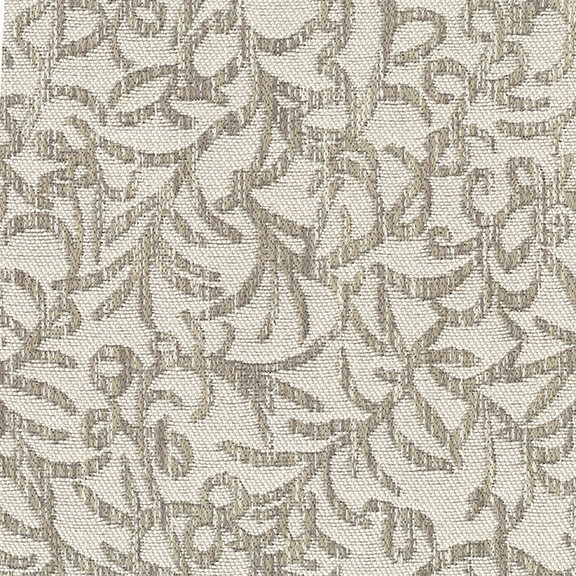This detailed color photograph showcases a textured fabric, possibly a quilted bedspread or a rug, featuring intricate embroidered patterns. The fabric itself is a neutral cream, light gray, or light brown shade, creating a subdued backdrop that accentuates the detailed embroidery. The embroidered designs, which resemble a series of intertwining leaves or tree branches, cover the fabric uniformly. These patterns appear in shades of grayish-tan or light tan, standing out against the lighter base. Some branches and leaves form circular or swirling arrangements, adding to the visual complexity. The uniformity and precision of the embroidery suggest it might have been machine-sewn rather than hand-stitched.